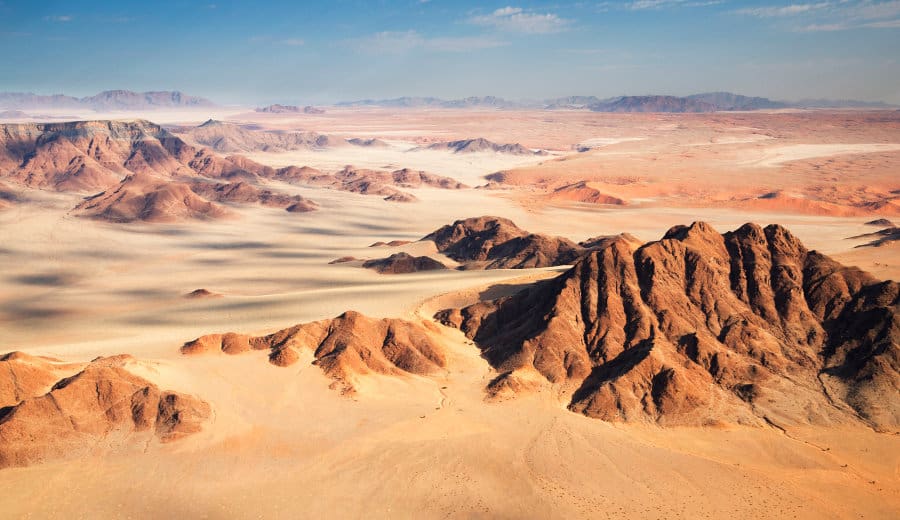This photograph captures a striking desert landscape featuring expansive stretches of golden and white sand, with distinct sand dunes reminiscent of small mountains. The foreground is dominated by golden-hued sand interspersed with rocky, hilly areas of a similar golden brown tone, which become taller and more pronounced on the right side of the image. Towards the center, the sand appears yellower, while the left side showcases patches of whitish sand speckled with black. The upper right background reveals a flatter, orangey terrain streaked with white sand spots, contrasting with the left side's craggy, brown rock-faced mountains. Farther into the horizon, darker, rugged mountains stretch across the skyline, intersected by reddish-brown mountainous regions that intertwine with the sand. The sky above is beautifully gradated from light to dark blue, darker on the left, and adorned with scattered, fluffy white clouds. Shadows cast by the mountains accentuate the depth and texture of this stunning desert scene.